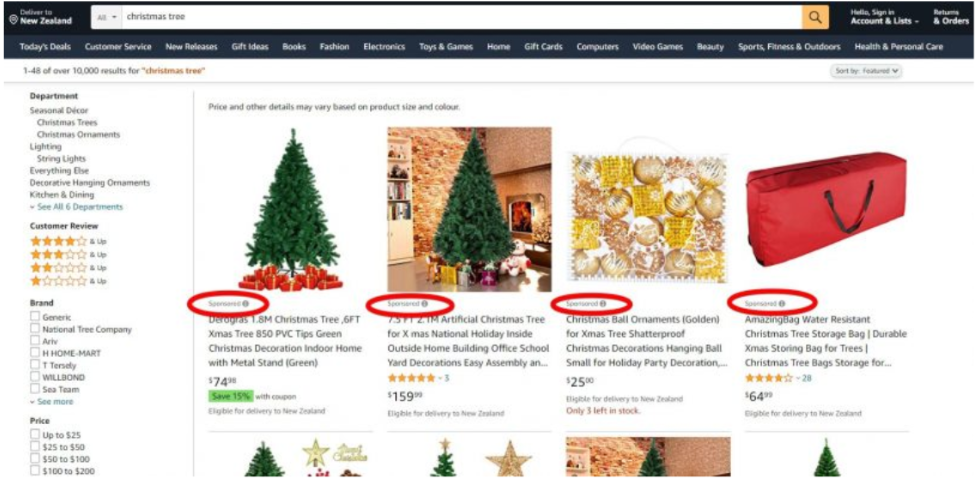This screenshot captures an Amazon webpage featuring a search results page for Christmas-themed products. The familiar black navigation banner is visible at the top, encompassing the search bar and a series of additional navigation options beneath it. Along the left-hand side, a sidebar provides further navigation choices such as department categories, customer reviews, and price filters.

The font in the screenshot appears tiny and somewhat difficult to read. Four main product thumbnails are prominently displayed on the results page. The first thumbnail on the left showcases a Christmas tree set against a white background, adorned with red gift boxes underneath. The second thumbnail also features a Christmas tree but is set in a cozy living room with multicolored gifts at its base. The third thumbnail is a photograph of various ornaments in shades of gold, copper, yellow, and silver. The final thumbnail displays a red Christmas tree storage bag.

Underneath each thumbnail, a thick red line highlights a specific detail, possibly circling the product's rating or price. Although the next four thumbnails are partially cut off, they also seem to depict Christmas trees, indicating a consistent theme in the search results.